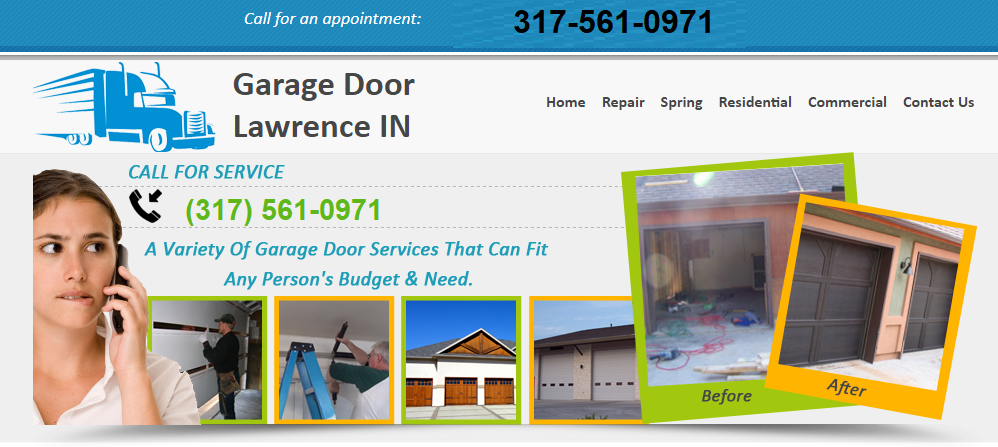This detailed image showcases a portion of a website dedicated to garage door services. At the top, on a blue background, there is an invitation to "Call for an Appointment" displayed in white text on the left side, while the right side features a phone number in black text. Below this header, the prominent title "Garage Door Lawrence IN" indicates the services are for Lawrence, Indiana. 

Adjacent to the title, on the left, is an animated image of a blue and white 18-wheeler truck, and to the right are six navigational categories laid out from left to right: Home, Repair, Spring, Residential, Commercial, and Contact Us.

Further down, on the left side, a call to action "Call for Service" is highlighted in blue text, accompanied by a black cell phone icon and a green phone number. Beneath this, blue text informs viewers about a variety of garage door services that can accommodate any budget and need. The segment displays a photo of a woman on the phone to the left, followed by two images of contractors at work, and two images of newly installed garage doors. 

On the right side, a green outlined square labeled "Before" is juxtaposed against a smaller, orangish-yellow square labeled "After," showcasing brand new dark brown garage doors.

The lower half of the image features a light gray background, completing the design and neatly organizing all the informational elements from top to bottom.